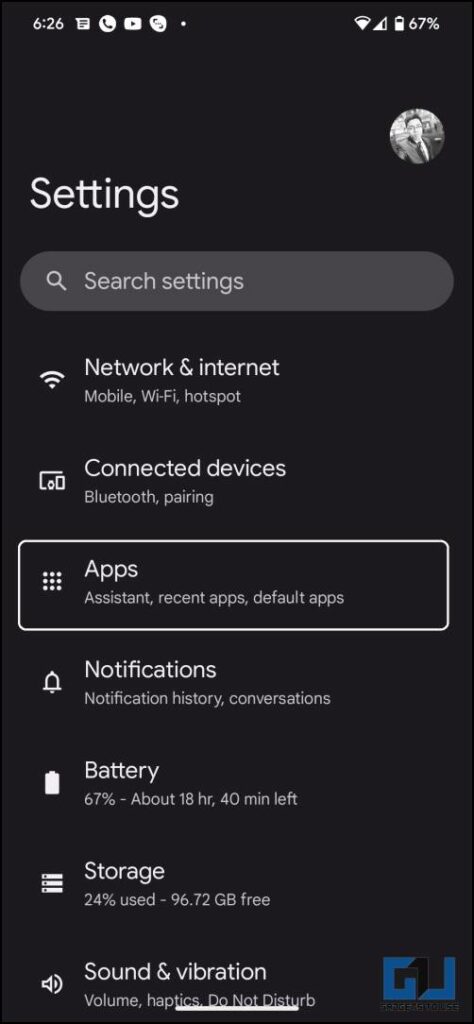This image appears to depict a smartphone's settings screen, likely used as the background for someone's phone. The background is solid black, and in the top left corner, the time is displayed as 6:26. Moving to the right, the battery level shows 67%. 

Underneath the battery icon on the right side, there is a profile picture icon that resembles an image of a male. Returning to the left, the word "Settings" is prominently displayed. Just beneath this, there is a grayscale search bar. Further down, a Wi-Fi icon indicates "Network and Internet" options, including "Mobile Wi-Fi Hotspot."

The next section lists "Connected Devices" with a Bluetooth pairing option. Following this, there are groups of small dots arranged in a 3x3 grid, labeled "Apps, Assistant, Recent Apps, Default Apps," each outlined in white. 

A bell icon signifies the notifications section, which includes "Notification History" and "Conversations." Another battery icon shows the current battery level again at 67%, with an estimated usage time of about 18 hours and 40 minutes left.

A second grid of small dots (3x3) is labeled "Storage," showing 24% used and 96.72 GB free. Following this is a speaker icon indicating "Sound and Vibration" settings, including volume, haptics, and a "Do Not Disturb" option. Finally, in the very bottom right corner, two blue initials "G" and "J" are displayed.